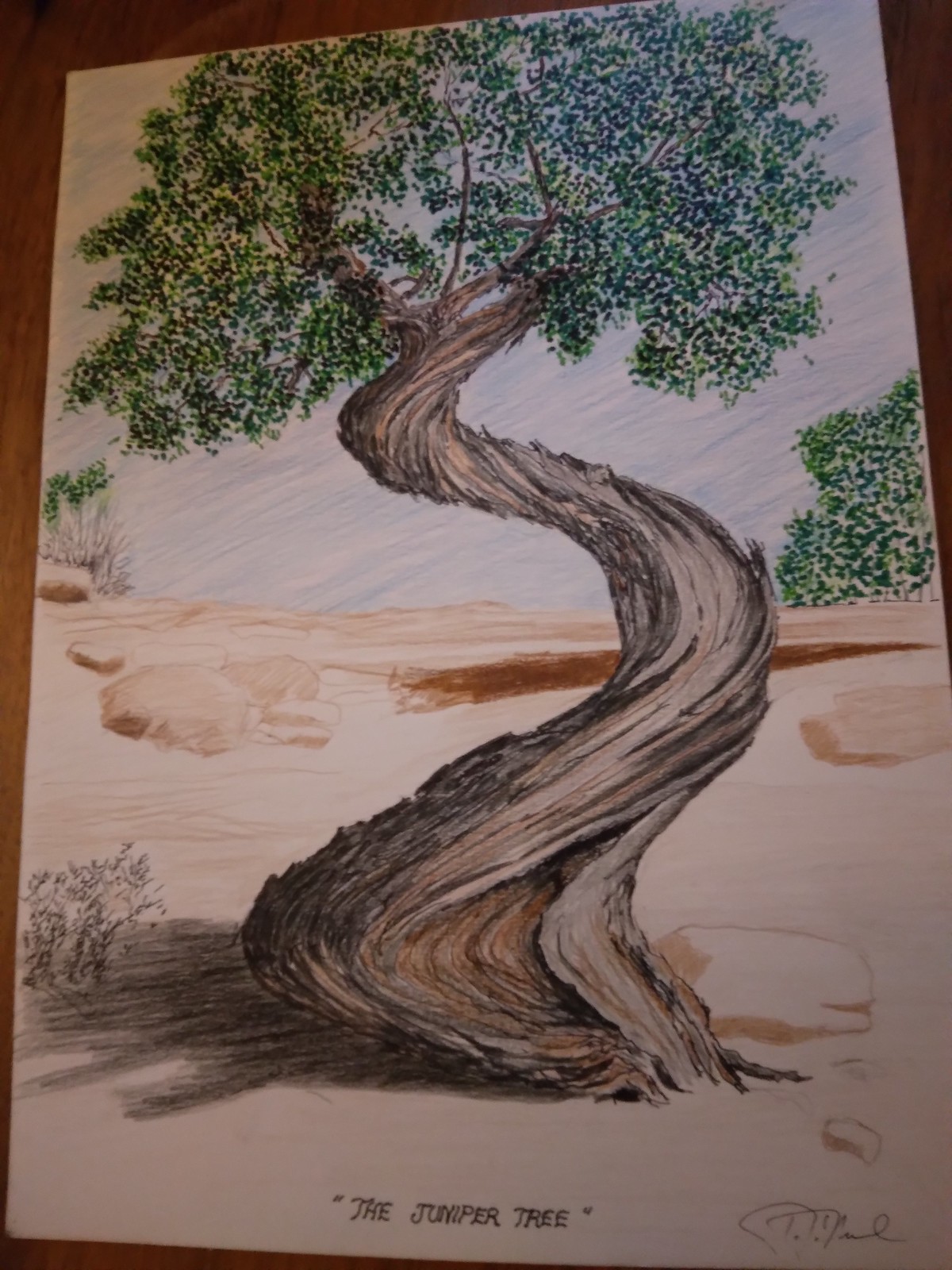This is a hand-crafted artwork depicting a juniper tree, as indicated by the black font inscription, "The Juniper Tree," at the bottom of the image. The artist's cursive signature is also present at the bottom. Dominating the picture is a brown tree with a uniquely twisted, spiral-patterned trunk set against a desert landscape. The tree trunk is a rich brown, and it casts a pronounced shadow on the tan-colored sand, which includes visible rocks, adding texture to the scene. The top of the tree is thick and lush with vibrant green leaves. Another tree with equally green foliage can be seen in the background among more rocks. The sky is represented through delicate blue shading, giving a serene backdrop to the detailed and dynamic desert scene.